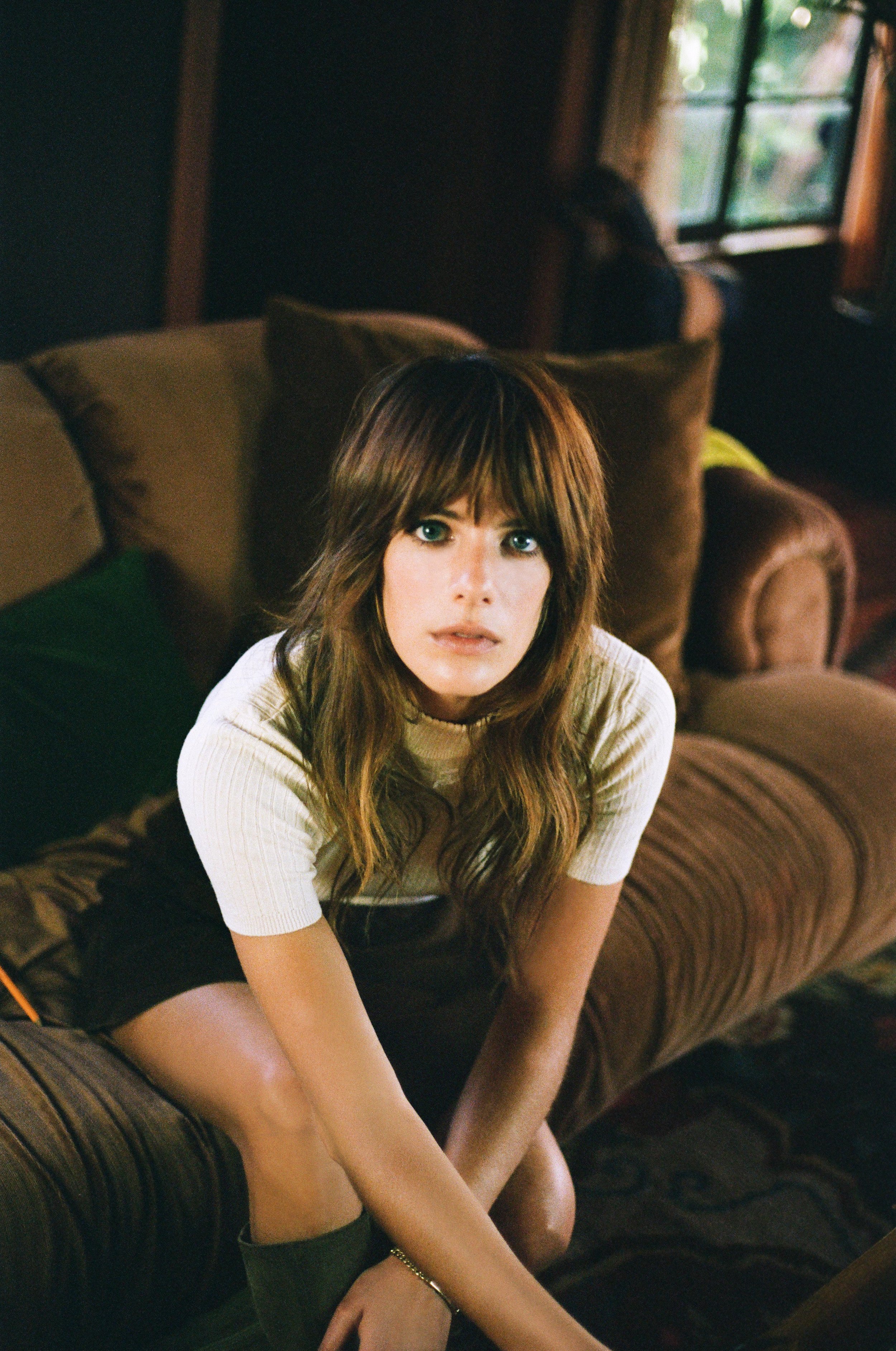In the image, a young Caucasian woman in her 20s or 30s is seated on a low, dark brown suede or velvet couch in a living room. She is positioned slightly forward, with her elbows resting on her knees and her arms crossed in an 'X' shape in front of her. Behind her are soft, smooth pillows that match the material of the couch. She wears knee-high black boots, a short black skirt, and a white ribbed short-sleeved t-shirt. Her long auburn hair flows past her shoulders, with bangs that nearly reach her blue eyes. She has pink lips and a thin silver bracelet on one arm. The room has visible light coming from a window to her right, which also offers a view of some greenery outside. The woman gazes inquisitively up at the camera, her expression a mix of curiosity and subtle worry. The ambiance is subtly illuminated by natural light streaming in from the window, highlighting the scene softly.